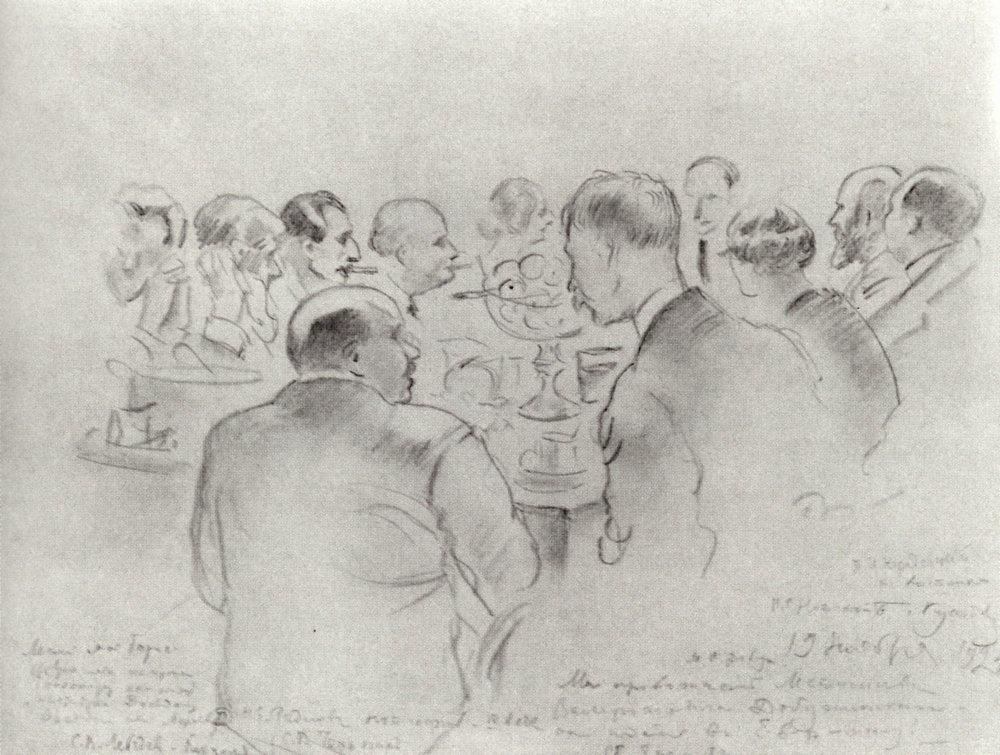This intricately detailed drawing depicts a diverse group of predominantly bald or balding men, along with two women, gathered around a table indoors, possibly for a business or political meeting. The scene captures a moment of interaction with most individuals’ attention directed towards the left of the frame. In the foreground sits a bald man, prominent and noticeable with his position. To his left stands or sits a thinner man with some hair and a mustache. Adjacent to him is a woman with a short haircut, adding a touch of gender diversity to the scene. Further along, two more bald men, one bearded, are engaged in the gathering. Among the group, a man wearing a tie with a mustache and another woman shown in profile stand out.

Central to the table is a bowl, possibly filled with fruit, perhaps apples, adding a semblance of a casual or break-time feel amidst the meeting. The detailed sketch highlights facial expressions and postures meticulously, noting even the subtlety of men smoking and another with his hands against his face.

The attire is formal, with visible suit coats among the men, which may signify the seriousness or formal nature of the occasion. At the bottom of the drawing, there is illegible cursive text, adding an authentic touch of handwritten detail which remains unreadable but atmospheric, suggesting a note or commentary related to the scene.